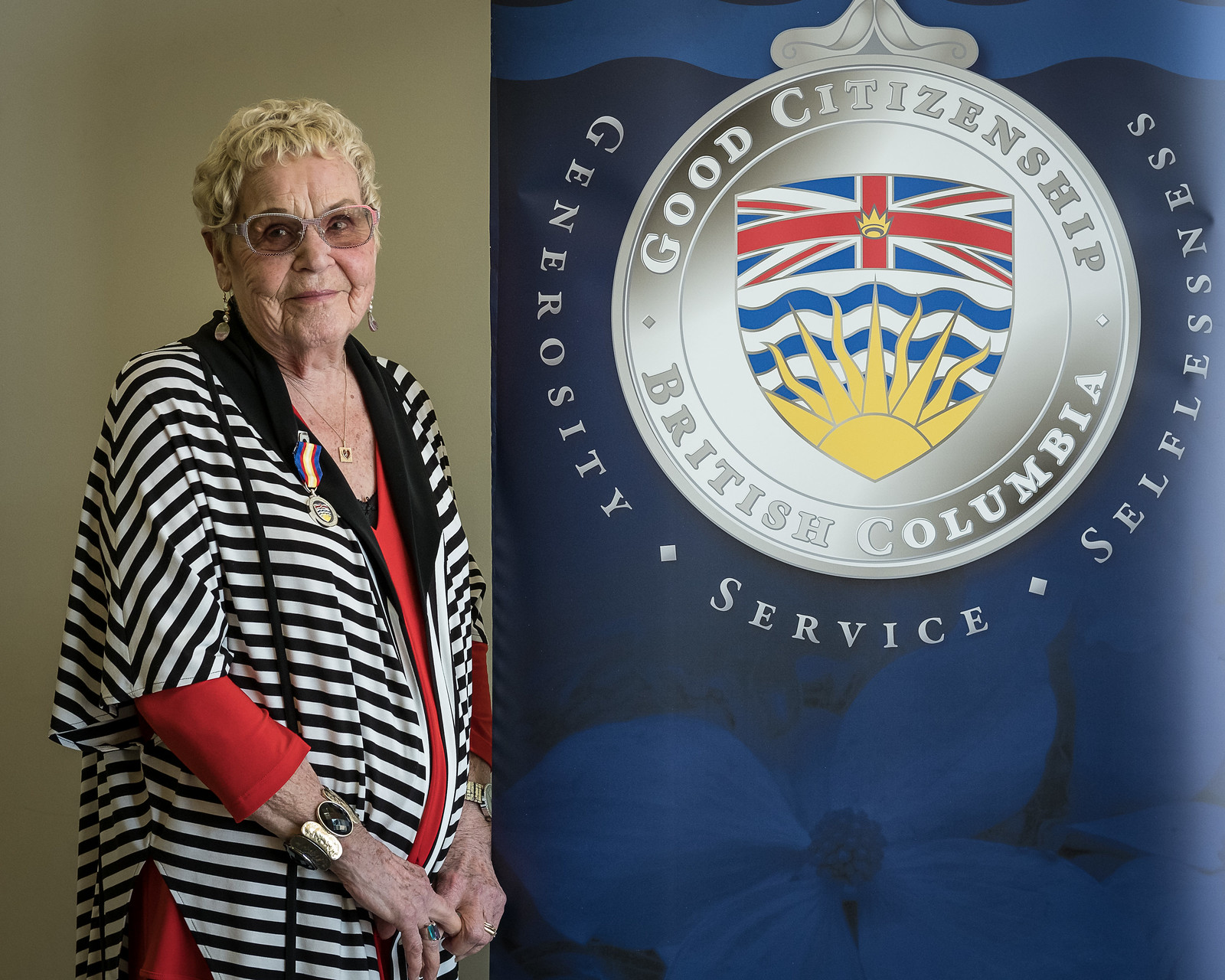A woman with short, blonde hair stands smiling against a tan wall on the left-hand side of the image. She wears dark-framed glasses with white and red edges on the sides, and a necklace featuring a small, square pendant. Her attire consists of a black and white striped jacket draped over a red shirt. On the upper left side of her jacket, she has an award medal pinned, and she also wears bracelets on both arms. To her right is a floor-length blue banner with a lighter blue flower near the bottom. In the middle of the banner, a silver medal is prominently displayed, inscribed with "Good Citizenship" at the top and "British Columbia" below. The medal includes an emblem resembling the British Columbia flag flanked by wavy white and blue lines with a sun beneath them. Surrounding the medal, in silver letters, are the words "Generosity," "Service," and "Selflessness." This image captures the woman being honored for her contributions to good citizenship in British Columbia.